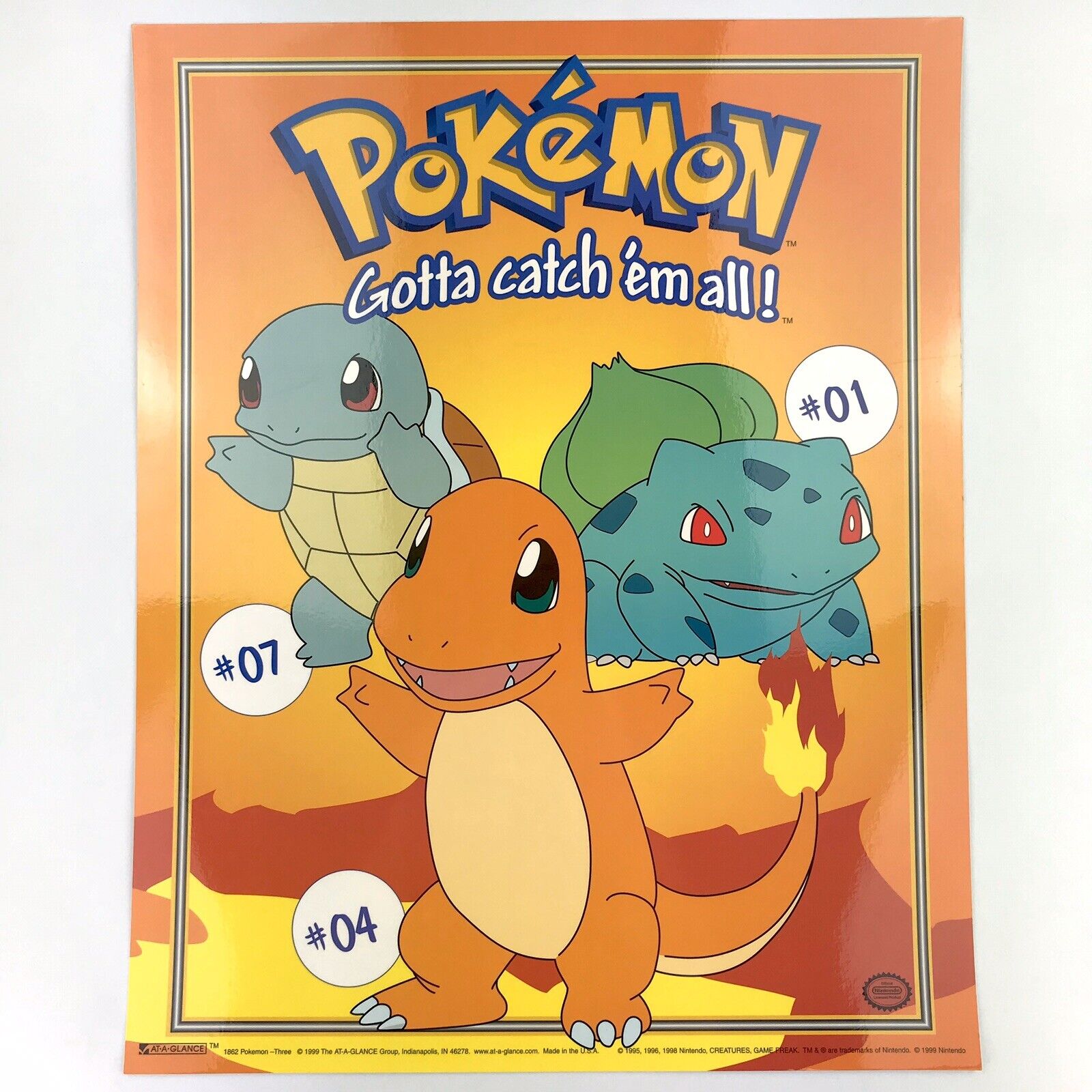The front cover of the Pokémon magazine features a vibrant orange background, prominently displaying the classic tagline "Pokémon: Gotta Catch 'Em All!" at the top. Central to the cover is Charizard, an orange dinosaur-like Pokémon with a beige belly and a flaming tail, labeled with a white circle containing the number 4. Flanking Charizard to the left, towards the back, is Squirtle, a small turtle Pokémon with a grey body and a brown shell, marked with the number 7 near its foot. On Charizard's right and slightly behind is Bulbasaur, a blue frog-like Pokémon with darker blue spots, red eyes, and what looks like a green garlic clove on its back; it bears the number 01. All three characters are depicted with cheerful expressions. Additional design elements include lines around the edges and some small, unreadable writing at the bottom.